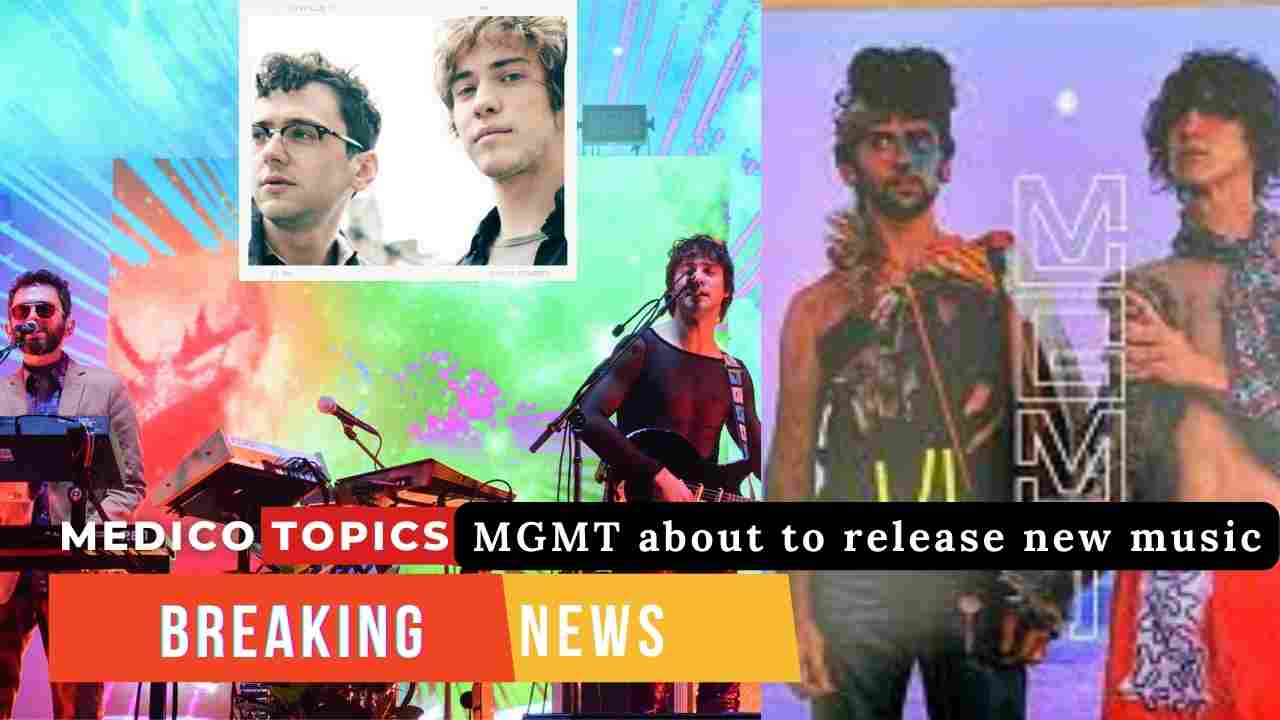This advertisement, possibly a poster or digital display, features the independent band "Medico Topics." The layout consists of three images of the two young male band members in different contexts. In the upper section, there's an inset close-up of both men's faces, with one wearing glasses and the other not. Below and to the left, another image captures them performing live on stage, with one handling a guitar and microphone, and the stage bathed in bright colors like purple, green, orange, and red. On the right side, a stylized photograph shows them in eccentric stage costumes and unconventional outfits designed to draw attention, set against a faint purple backdrop. This section includes vertical text reading "MGMT."

The promotional text is scattered throughout the display. At the lower third, bold script reads, "Medico Topics Management about to release new music. Breaking News," where "Breaking" is set against a white background and "News" against an orange-tan background. The overall aesthetic of the advertisement suggests amateur, self-made credentials, characteristic of an independent band.